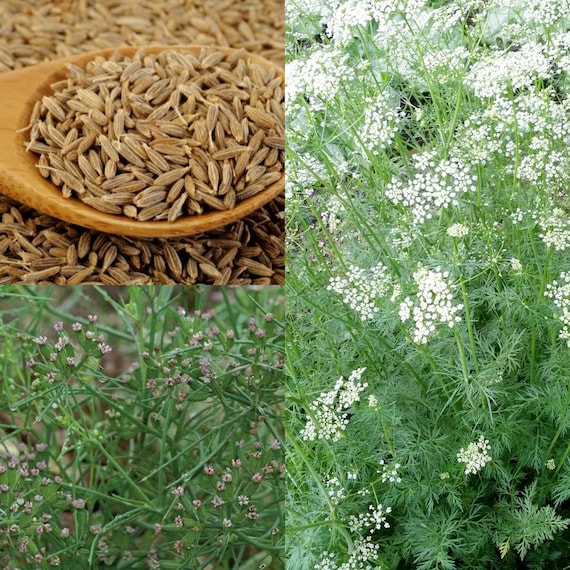The image is a detailed composition of four smaller square images forming one larger square, reminiscent of a layout from a scientific textbook. The upper left image features a shallow, rounded wooden bowl filled with light and dark brown seeds, reminiscent of fennel seeds, scattered both inside and outside the bowl across the floor. Moving clockwise to the upper right image, we see a dense, full-screen view of grey foliage with numerous stems and spiky leaves, sporadically dotted with very tiny white clusters of flowers or buds. The lower right image presents a close-up of thin green stalks and leaves dominated by minute pink flowers, covering the entire frame. Lastly, the lower left image provides a ground-level perspective of greenery with thin stalks and occasional tiny flowers, harmoniously filling the picture.